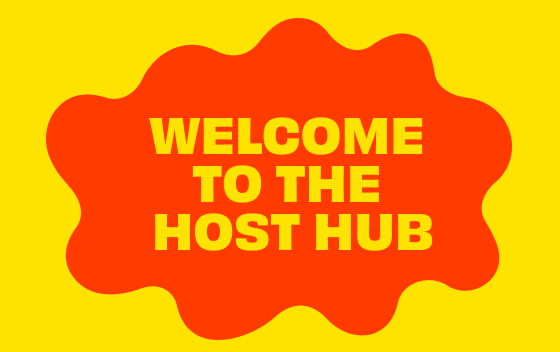The image is a digital poster with a bright yellow rectangular background. At the center of the image is a prominent, wavy, red splatter resembling a blob of paint. Within this red splatter, there is yellow text arranged in three rows. The text reads: "Welcome" on the first row, "to the" on the second row, and "Host Hub" on the third row. The entire design is simple and cartoon-like, with only two colors—yellow and red—used throughout. The layout is straightforward, featuring upright objects and a clear, digital quality that suggests it could have been professionally designed.